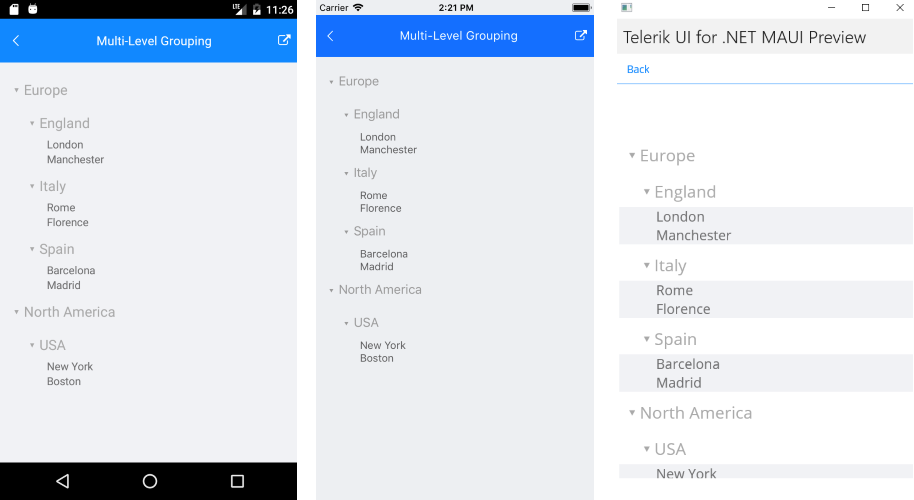The images present a side-by-side comparison of three screenshots, likely taken from mobile phones, showcasing various levels of content hierarchy.

1. **First Image**: 
    - **Header**: "Multi-level grouping"
    - **Region Labels**:
        - **Europe**:
            - England: London, Manchester
            - Italy: Rome, Florence
            - Spain: Barcelona, Madrid
        - **North America**:
            - USA: New York, Boston
    - **Additional Detail**: The top of the image displays signal strength indicators, suggesting it was taken from a mobile phone.

2. **Second Image**: 
    - **Header**: "Multi-level grouping"
    - **Region Labels**:
        - **Europe**:
            - England: London, Manchester
            - Italy: Rome, Florence
            - Spain: Barcelona, Madrid
        - **North America**:
            - USA: New York, Boston
    - **Additional Detail**: Similar to the first, this image shows battery life icons.

3. **Third Image**: 
    - **Header**: "Telerik UI for .NET MAUI Preview"
    - **Region Labels**:
        - **Europe**:
            - England: London, Manchester
            - Italy: Rome, Florence
            - Spain: Barcelona, Madrid
        - **North America**:
            - USA: New York, Boston
    - **Additional Detail**: Again, this image includes content hierarchy but under the Telerik UI branding.

The consistent labeling across the three images suggests they are demonstrating different implementations or presentations of the same data in various apps or perhaps different stages of design on mobile devices.